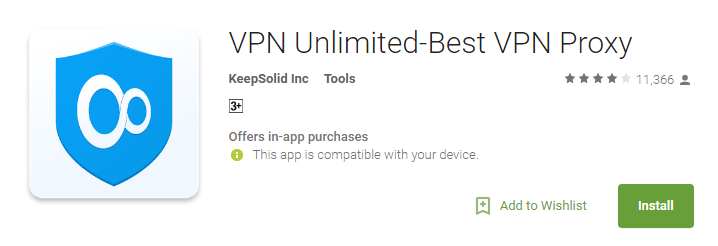The image displays a rectangular information bar with a white background, oriented horizontally rather than vertically. On the left side, there is a square section featuring a white background with a blue shield icon that contains a horizontally-positioned infinity symbol. Notably, the right circle of the infinity symbol is smaller than the left circle.

To the right of this icon, the text reads "VPN Unlimited - Best VPN Proxy." Below this, it is indicated that these tools are provided by "KeepSolid Inc."

Further right, the image displays a rating of four stars accompanied by 11,366 reviews. Below this rating, there is a label marking the app as suitable for ages 3 and up and noting that in-app purchases are available. 

The compatibility of the app with the user's device is also highlighted with text stating "This app is compatible with your device." Adjacent to this text, there is a green button featuring an eye icon.

Toward the far right, there's an "Add to wishlist" option represented by a green button with a banner or bookmark icon containing a plus symbol. Below it, a larger green button displays the word "Install" in white text. The overall color scheme of the image includes blue, green, black, and white elements.